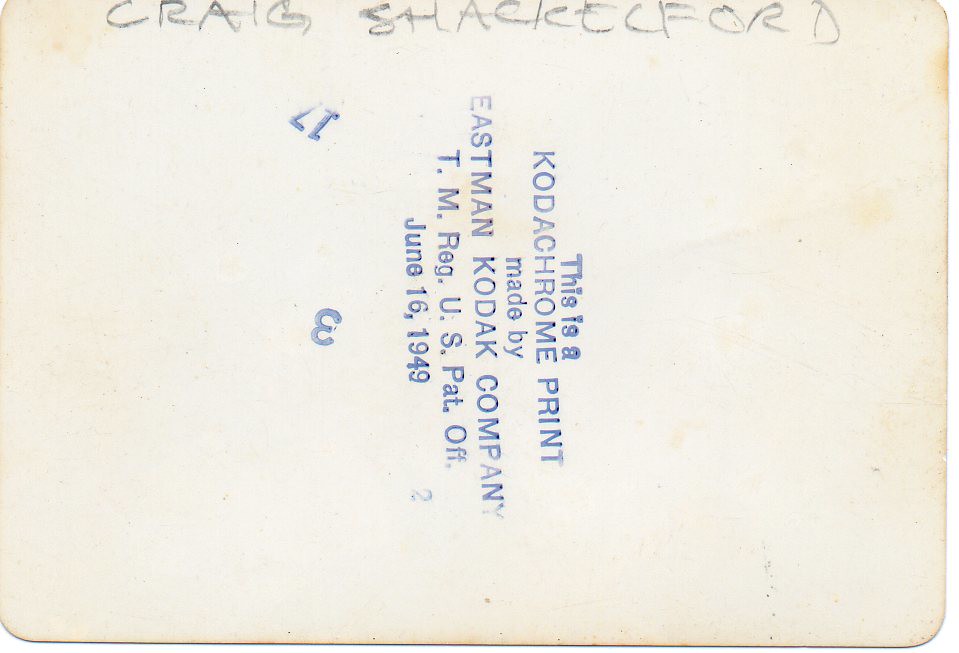The image features an aged piece of paper that appears to have originally been white but has since developed a yellowed or browned patina around its edges, indicative of its age. The central area of the paper remains relatively brighter and less aged. Positioned horizontally, the paper is oriented in a landscape format. At the top, the name "Craig Shackelford" is inscribed in pencil. Further down, there's a blueprint-like, stamped message which reads: "This is a Krotokome print made by Eastman Kodak Company, T.M. Reg. U.S. Pat. Off., June 16, 1949."